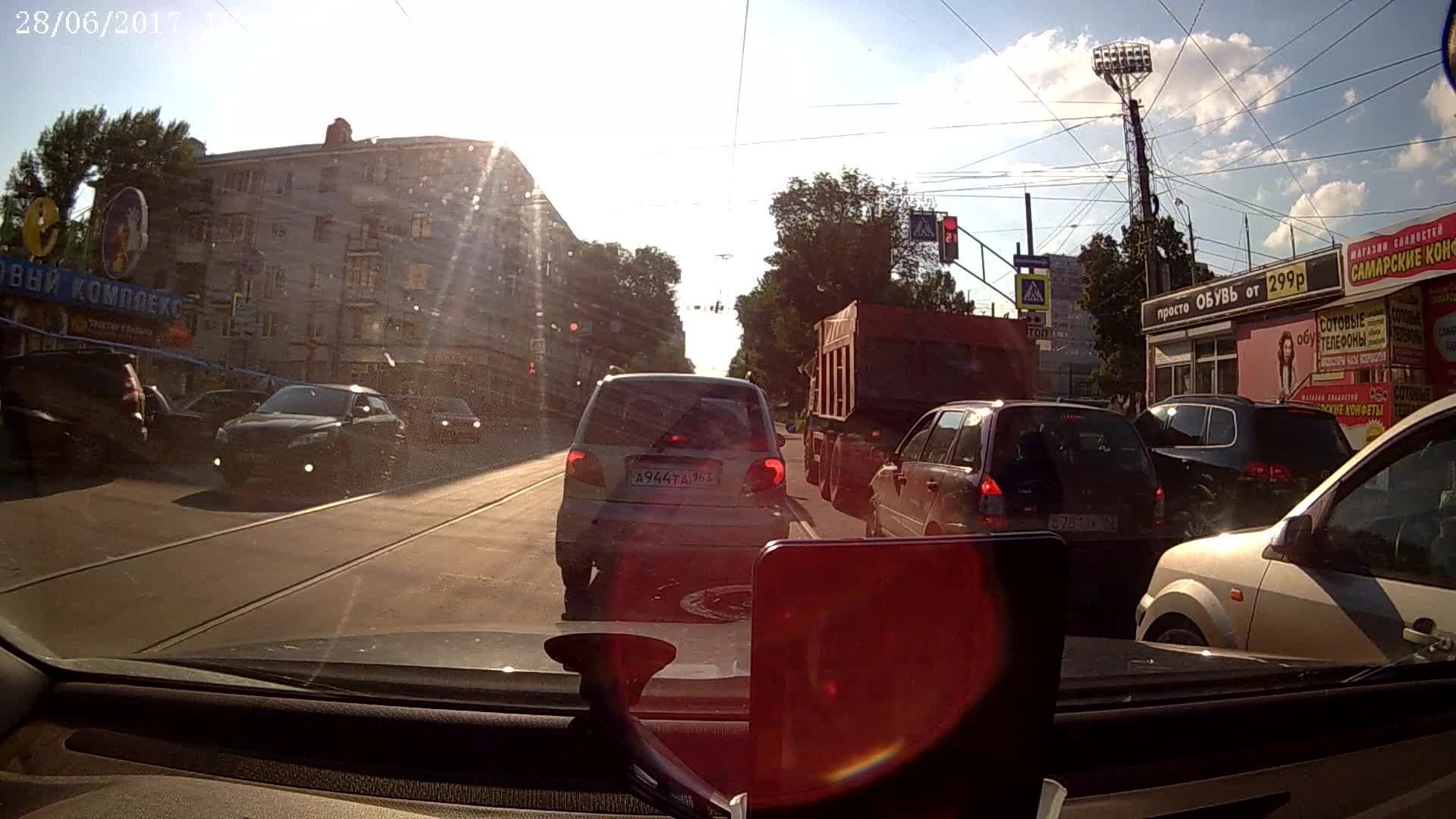The image depicts a vibrant scene in a small town, captured from inside a vehicle, possibly a bus, evidenced by the wider windshield and visible door handle. The clear, sunny day is punctuated with white, fluffy clouds decorating the blue sky. The street is bustling with traffic, including a gray SUV with red lights illuminated, a gray car, a black crossover vehicle, and several minivans, all positioned across three lanes of traffic. The road is lined with various buildings; to the left stands a tall, older-style gray building, possibly a hotel, with numerous windows. On the right side, there are stores that might be insurance offices or corner shops. Prominent in the background is a large radio or water tower, with verdant green trees interspersed throughout the scene. The sun casts a glare, especially noticeable on the silver minivan and the white vehicle. Electric lines crisscross the sky, enhancing the small-town atmosphere depicted in the photograph.